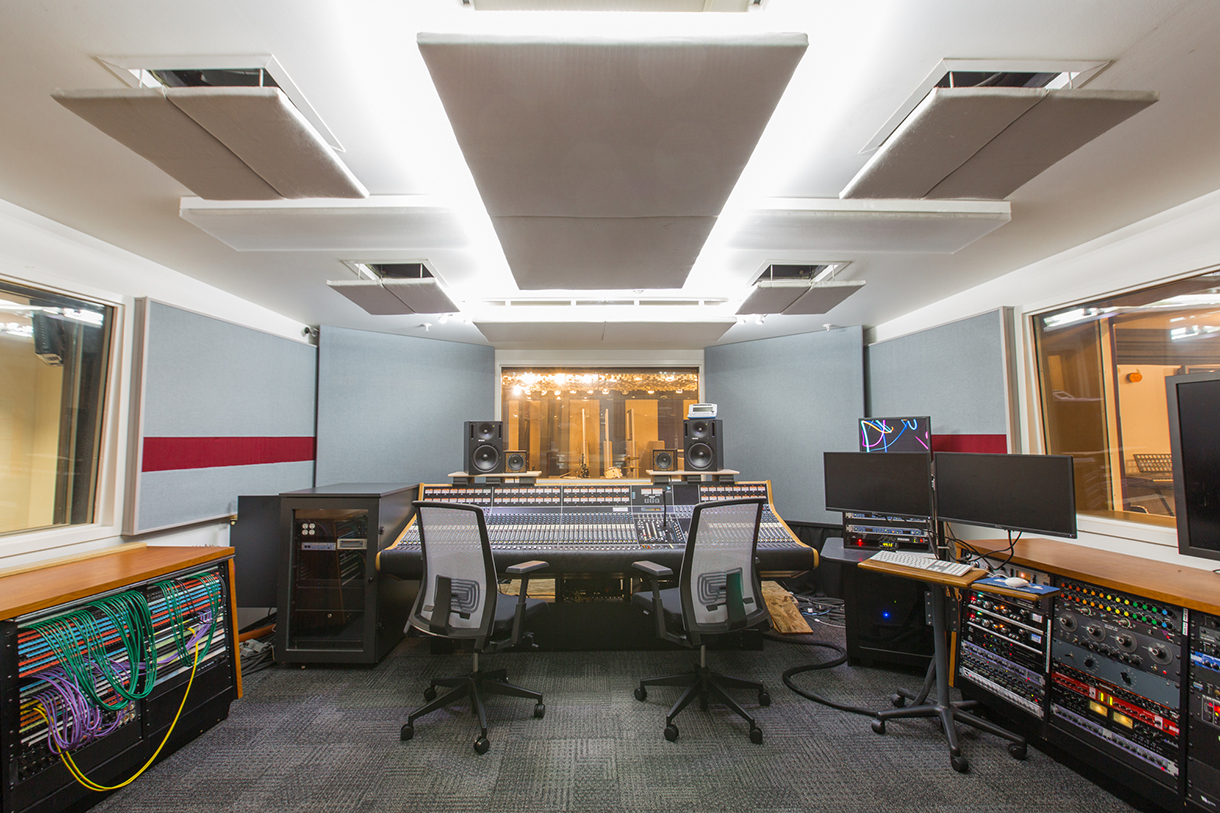The image depicts a sophisticated recording studio and control room, surrounded by large windows on three sides that offer views of the outside, including many tall buildings visible through the far-end window. The room features brown wooden shelves along both walls, which are equipped with numerous musical recorders and devices filled with buttons, knobs, and electrical components. In the center of the room, two black office chairs with white backs are positioned in front of a lengthy soundboard that has an abundance of knobs and buttons. On the walls, there are monitor speakers on either side, housed alongside other pieces of recording equipment and computer screens that aid in monitoring studio activities. The walls of the room are painted in a combination of gray and white with a red stripe, and the floor is covered with grayish carpet tiles. The ceiling includes several lights to illuminate the setup. The whole scene exudes the vibe of a powerful and comprehensive recording studio, tailored for creating and producing music.